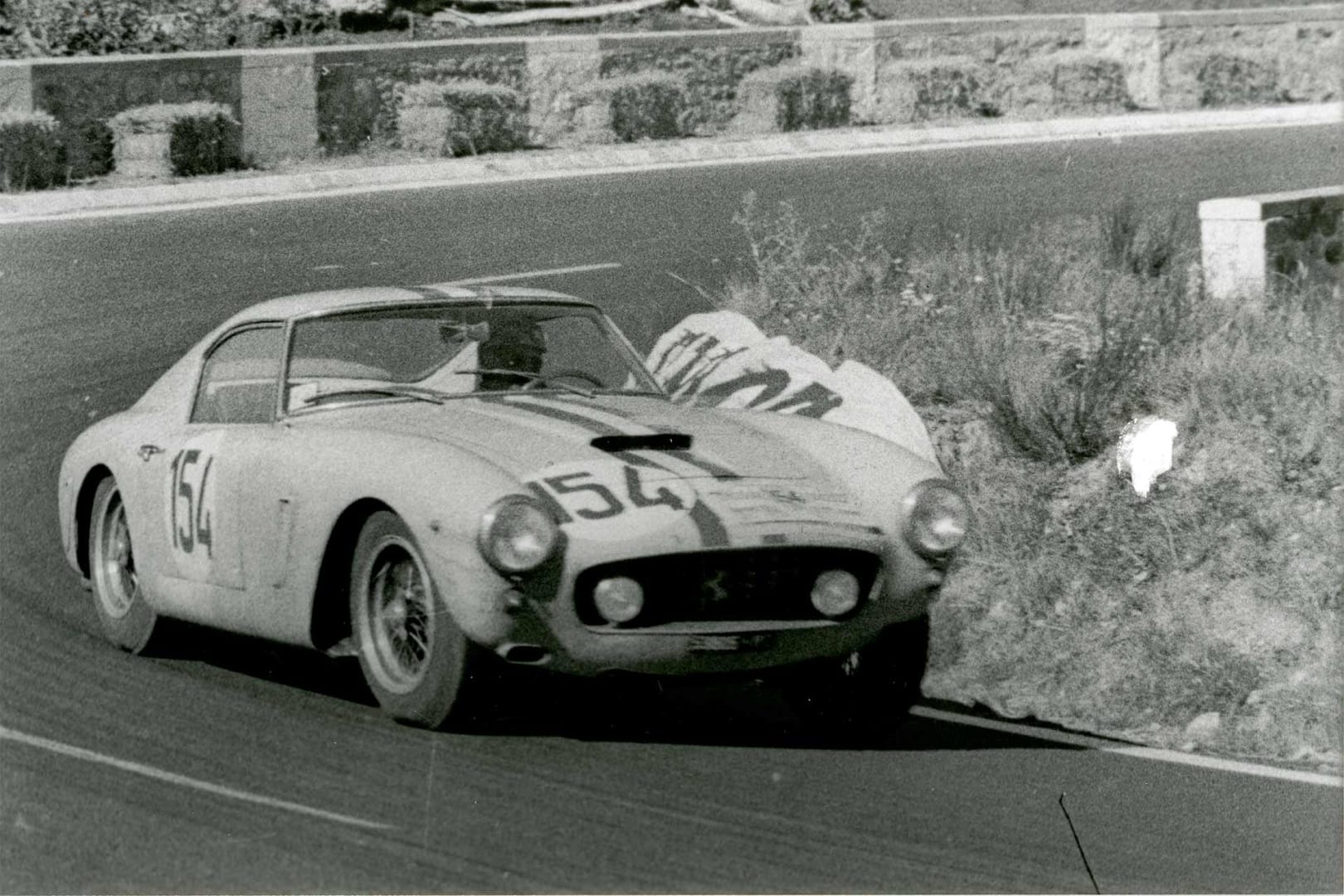This black-and-white photograph evokes a nostalgic, vintage feel, reminiscent of eras before the 2000s. Dominating the scene is a classic two-door race car with racing stripes, identified by the prominent number "154" painted on both the hood and the passenger side door. The car, potentially a Ford, is navigating a sharp U-turn on a curving road that enters the image from the top right, sweeps left, and exits at the bottom right. 

The driver, possibly a race car driver wearing a helmet, is partially obscured in the shadow. Surrounding the road are hay bales and a sparse, grass-filled field resembling a desert landscape. In the background, a small brick wall with a sidewalk runs alongside the road, lined with potted plants or bushes, adding to the vintage atmosphere. The image captures the car in mid-turn, heading towards the viewer, creating a dynamic sense of motion.